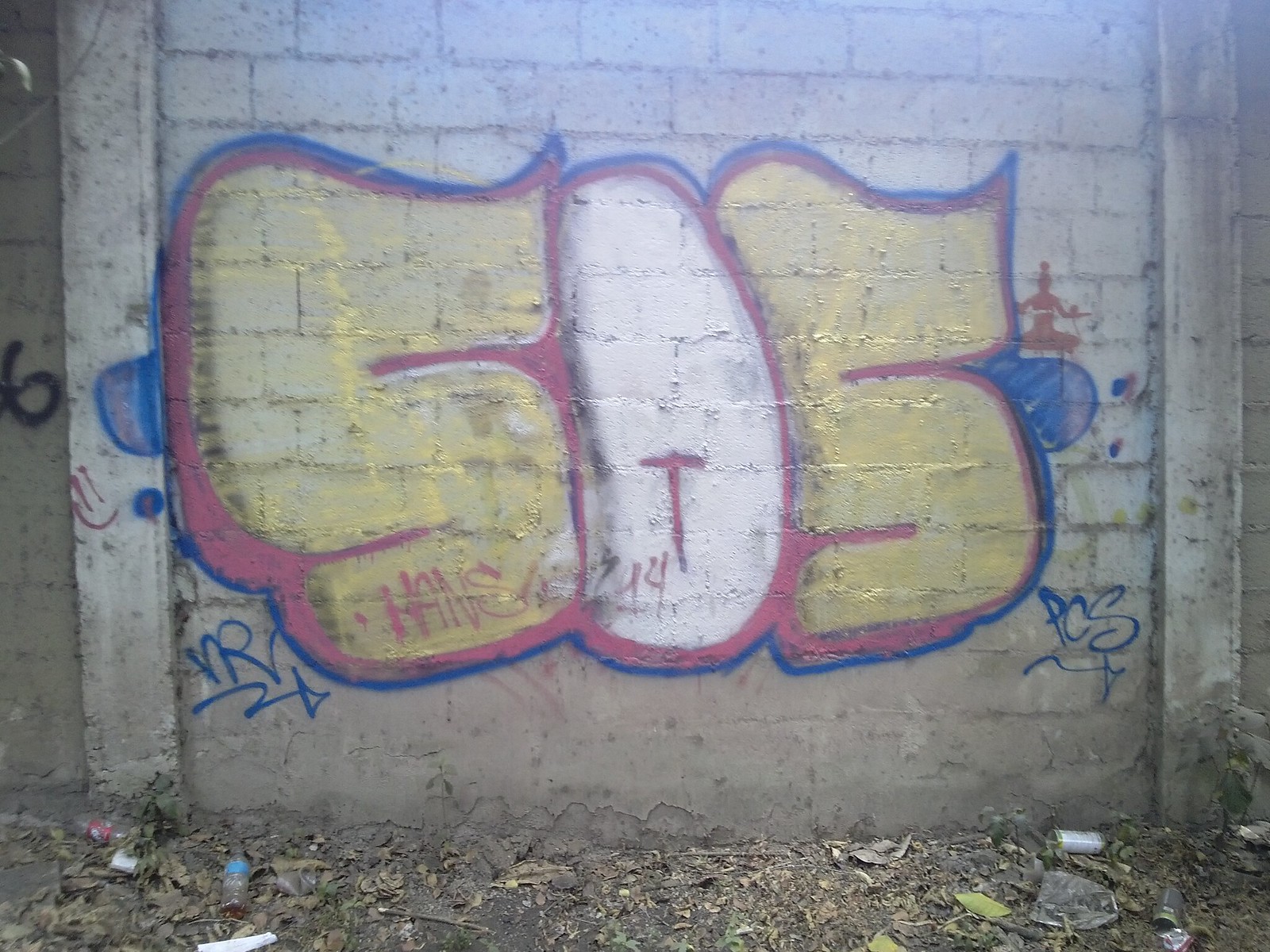The image shows a dilapidated, white-painted cinder block wall covered in graffiti. The ground in front of the wall is littered with trash, including empty spray cans, leaf litter, and bottles. The central graffiti piece displays the large letters "SOS," rendered in bubble lettering. The first 'S' and the last 'S' are painted yellow, each outlined in blue and pink. The first 'S' is further adorned with the name "HANS" inscribed in pink. The 'O' features a reddish 'T' in its center, with the number '14' just below it. Surrounding the graffiti are additional artistic elements: a blue blob extending from the last 'S', a small orange silhouette resembling a meditating figure, the initials 'PCS' in blue at the bottom right, and 'VR' along with a jagged arrow on the left. Additionally, the far left of the wall bears the spray-painted number '6' in blue. The overall setting is dreary and neglected, enhancing the gritty aesthetic of the urban artwork.